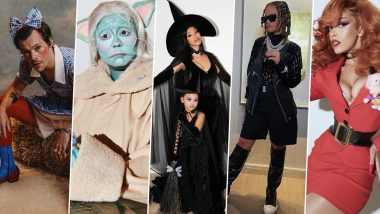This series of five vertical images showcases various elaborate Halloween costumes. On the far left, a man kneels in an extravagant Ace Ventura ensemble, complete with a blue bow in his hair, a blue and white printed shirt, red tights, and blue socks. His right hand covers his ear while the left hand hangs down. To his right, a person embodies Yoda, their face painted green with large pointy ears, featuring pink inner ear detailing. They don a tan robe-like jacket. Continuing rightward, an older woman and a young girl are both attired as witches. The older woman wears a grand black witch hat, a witch gown, and dark gloves, while the young girl matches in a smaller witch hat and black dress, holding a broomstick. Adjacent to them is a woman sporting dark sunglasses, a black trench coat, black shorts, pearl necklace, long socks, and white shoes. Further right, a woman with bright red hair stands confidently in a tight red dress just above her thighs. She accents the outfit with a wide black belt and red lipstick. Her right hand is raised, and a small doll of an old man is pinned to her shoulder. Each costume reflects detailed creativity, making the collection a lively celebration of Halloween.